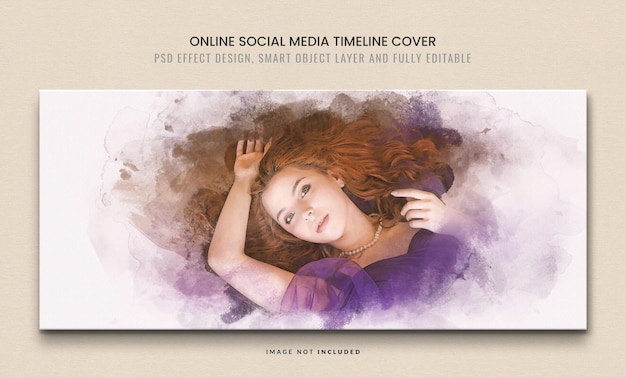The image depicted is a horizontally long, vertically short painting used as an example for an online social media timeline cover. The background is a pristine white canvas, featuring a young, fair-skinned woman with flowing, wavy red hair spread around her as she lays on her back. She is adorned in an elegant, poofy purple chiffon-like dress with short, sheer sleeves and a low neckline. One of her arms is gracefully raised above her head, while her other hand rests below her chin, partially within the cascade of her hair. Around her neck, she wears a white pearl choker necklace. The background of the canvas is also embellished with a purple mist or cloudy effect, which intricately surrounds the woman. In black text near the top, the canvas reads "online social media timeline cover," and below that in gray text, it states "PSD, effect design, smart object layer, fully editable." At the very bottom, in small print, it notes "image not included."